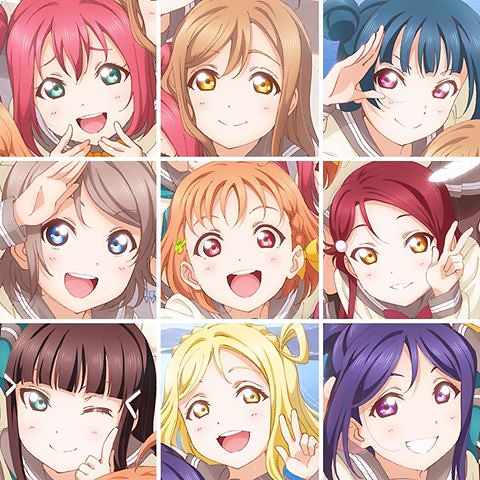The image is a grid of nine evenly spaced cartoon illustrations of anime-style girls, each occupying one of nine neatly arranged squares (three per row). Each girl has distinct hair and eye colors, as well as different poses and expressions. From left to right, starting at the top: the first girl has red hair and green eyes, the second has brown hair and yellow eyes, and the third has blue hair and pink eyes. The middle row features a girl with brown hair and blue eyes, followed by one with orange hair and red eyes, and another with red hair and orange eyes. The bottom row shows a brown-haired girl with green eyes, then a blonde girl with yellow eyes, and finally a girl with purple hair and pink eyes. All the girls are smiling or laughing, exuding a cheerful and cute demeanor, and several are striking playful poses such as saluting, waving, or making a peace sign. Some details like freckles further enhance their unique and adorable appearances.